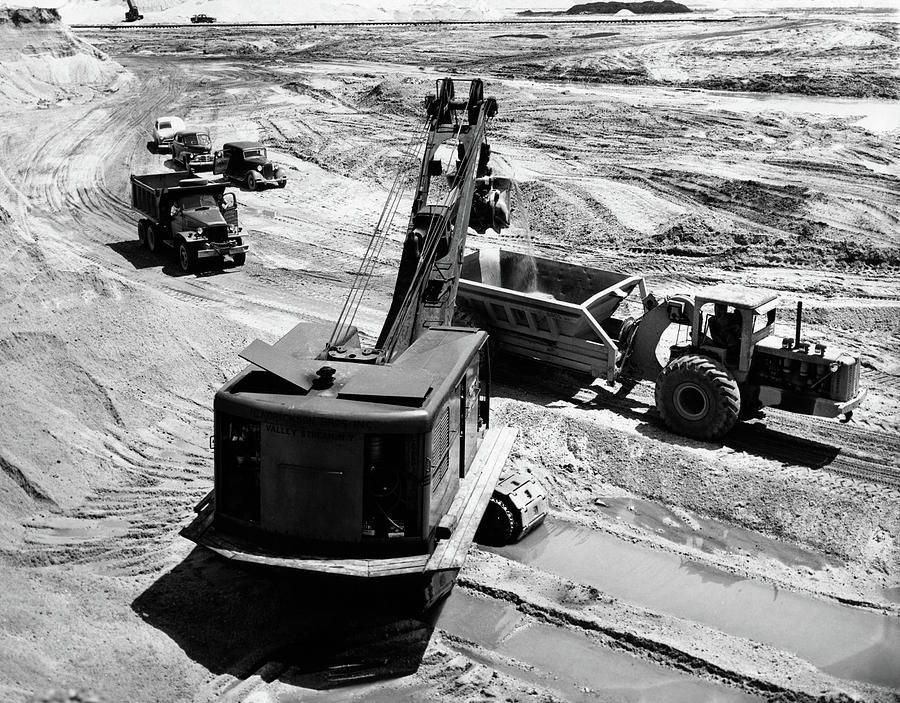This black-and-white photograph, likely dating from the 1920s to 1950s, captures an active construction site in a desert-like, dirt-filled area under bright, sunny skies. The image, presented in a square format from a slight aerial perspective, focuses on several pieces of heavy machinery, including a bulldozer, a crane, and a large tractor-like vehicle with a dump truck portion. These vehicles are busy working the surface, leaving visible textured markings from their wheels. The central piece of equipment faces away from the viewer. In the far distance, more machinery can be seen approaching. Old vehicles, characteristic of the 1930s to 1940s, are visible on the left side, adding historical context to the scene. Notably, the writing on one truck indicates a company name with "Valley" and suggests the transportation of materials like sand for what appears to be roadway construction.